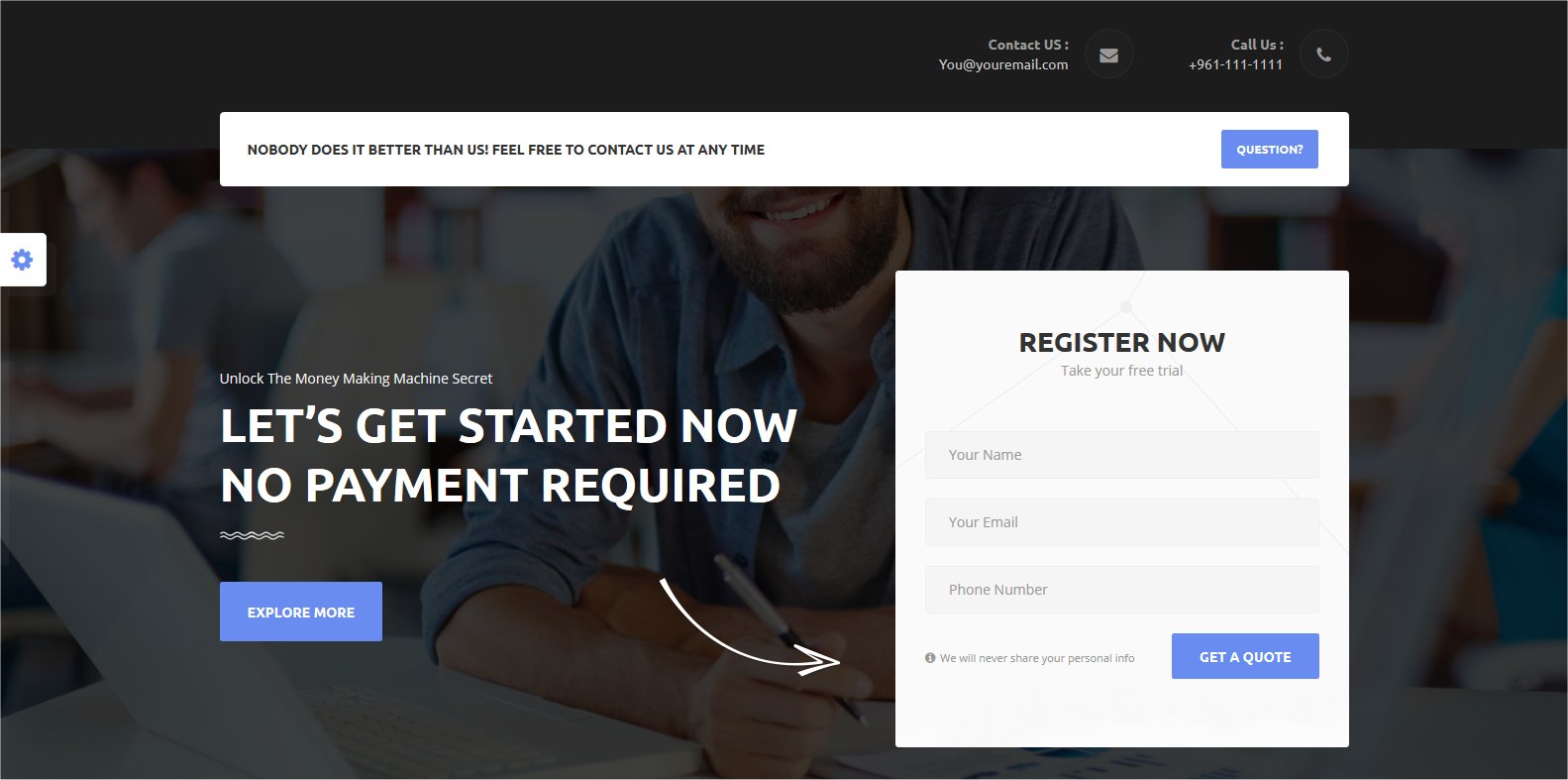The image depicts a cell phone screen showcasing a sales landing page with a predominantly black background. This image, wider than it is tall, appears to be captured from a computer display. 

The upper section of the screen features a solid black rectangle with a visually striking image underneath it. This image shows a man holding a pen in his right hand, partially obscured by a blue or black overlay. Adjacent to this image, there is a prominent white box with the text: "Nobody does it better than us. Feel free to contact us at any time." Below this, more contact information is listed: "You at youremail.com" and "Call us: 961-111-1111."

On the lower left-hand side of the screen, the phrase "Unlock the Money-Making Machine Secret" is displayed. Below this, in larger uppercase white font, it says, "LET'S GET STARTED NOW, NO PAYMENT REQUIRED." This text is accompanied by wavy lines and a blue button with white text that reads "EXPLORE MORE."

The right section of the bottom half encourages users to "REGISTER NOW," featuring a white arrow directing attention from the left-side content to a registration form. This form asks for the user's name, email, and phone number, promoting a "FREE TRIAL" and offering to "GET A QUOTE."

The overall tone of the page is very promotional and infomercial-like, typical of landing pages designed to capture leads after a free webinar or similar introductory event.